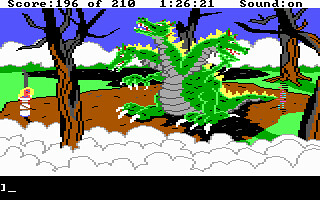The screenshot of the video game features a detailed overlay across the top, displaying the score "196 of 210," the time "1:26:21," and "Sound: On" in black lettering. At the bottom, a black band frames the scene. The background showcases a bright blue sky adorned with a line of white clouds stretching horizontally. Below, lush green grass extends across the landscape, interrupted by a black patch from which leafless trees, colored in shades of brown, black, and gray, emerge. Dominating the scene's center is a formidable three-headed dragon with a green body, a gray belly, two feet capped with white toenails, and a long green tail lined with yellow bumps. Each of its heads also sports yellow bumps along the back. Positioned on the far left stands a girl, seemingly bound to a rod, with white puffy material below her, potentially a cloudy mist or part of her attire.